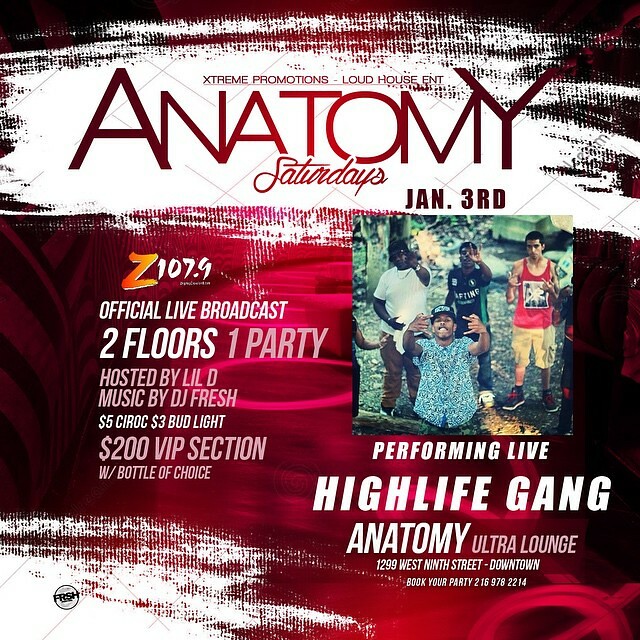The image is a detailed flyer promoting a club event by Extreme Promotions and Loud House Entertainment, titled "Anatomy Saturdays," taking place on January 3rd. The flyer has a predominantly red background with white and pink elements. At the top, in bold red letters, it reads "Extreme Promotions Loud House Entertainment," followed by "Anatomy Saturdays" and the date "January 3rd." Below this header, there's a vibrant picture of four men posing and making various hand signs. 

To the left side, the text features the sponsor Z107.9, highlighted with an orange "Z", followed by "Official Live Broadcast." The flyer continues to detail the event with "2 Floors 1 Party," "Hosted by Lil D," and "Music by DJ Fresh." Prominent drink specials include "$5 Ciroc" and "$3 Bud Light." Additionally, it mentions a "$200 VIP Section with Bottle of Choice." 

On the right side, the flyer announces "Performing Live: High Life Gang," with a note that this event will be held at "Anatomy Ultra Lounge," located at "1299 West 9th Street Downtown." Contact information to book a party is also provided: "216-978-2214." The flyer is visually striking with a combination of white and black streaks against the red background, adding to its dynamic and energetic feel.